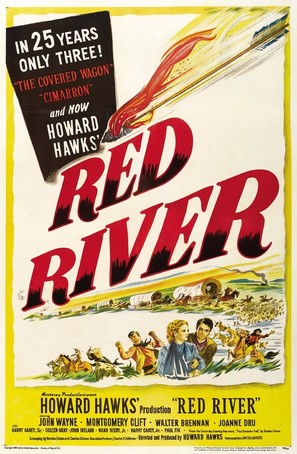This image depicts an intricately designed poster for the movie "Red River." The poster is bordered by a dark yellow edge. Dominating the central imagery is a covered wagon caravan accompanied by a dynamic scene featuring several people; some are running or possibly involved in a skirmish, and a few are mounted on horseback. Toward the top right-hand corner, a flaming arrow streaks dramatically toward the center of the image.

At the top left of the poster, bold text reads: "In 25 years, only three. The Covered Wagon, Cimarron, and now Howard Hawks' Red River." Beneath this text, a striking illustration shows a man standing behind a blonde woman dressed in a blue jacket and scarf, as she looks over her left shoulder toward him.

Further down, prominently placed, are the movie’s title in big red letters: "Red River." Below the title, the poster credits this work as a Howard Hawks production and lists some of the starring actors, including John Wayne, Montgomery Clift, Walter Brennan, and Joanne Drew. Additional smaller text is present but is difficult to discern.